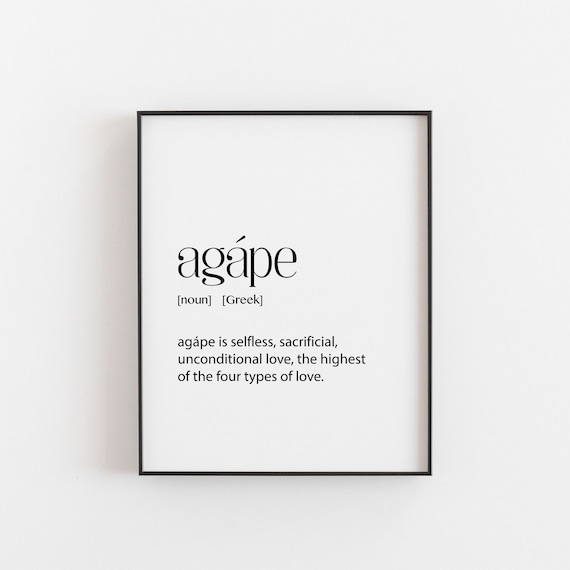The photograph depicts a minimalistic black and white framed text hung on a plain white wall with a faint grey gradient towards the bottom. The text inside the very thin black frame is a dictionary definition of the Greek word "agape." The word “agape” is prominently displayed in large black lowercase letters, with an accent mark over the first letter 'a', emphasizing its foreign origin. Below, in smaller text within brackets, it states "noun, Greek." The definition spans three lines, explaining that agape is "selfless, sacrificial, unconditional love, the highest of the four types of love." A subtle shadow of the frame falls towards the left, adding depth to the image. There are no other objects or distractions in the composition, allowing the viewer to focus entirely on the profound meaning of the word agape.